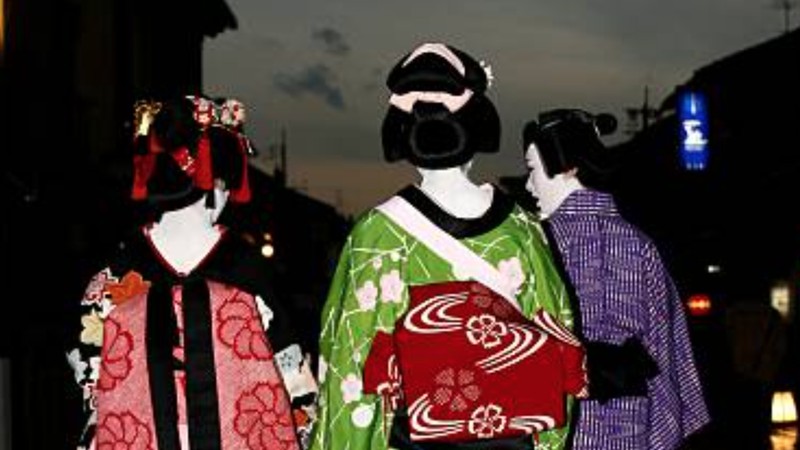The photograph, likely a digital painting, portrays a nocturnal urban scene featuring three individuals dressed as geishas. The figures are walking away from the camera, immersing viewers in their traditional Japanese attire. The leftmost figure dons a pink and black kimono, adorned with red tassels and flowers in her hair. The central figure wears a green flowered kimono, complemented by a red pack on her back and white detailing in her hair. The rightmost figure is clad in a striking purple striped kimono, paired with a black obi, and also decorated with flowers in her hair. Both their skin and that of a man to their right, wearing traditional Japanese garments, are painted white. The man glances slightly towards the observer, revealing part of his face. They traverse a dimly lit city street, flanked by indistinct buildings with hints of windows and neon signs. The sky above is a mix of dark green-gray hues tinged with red, suggesting the final moments of a sunset.